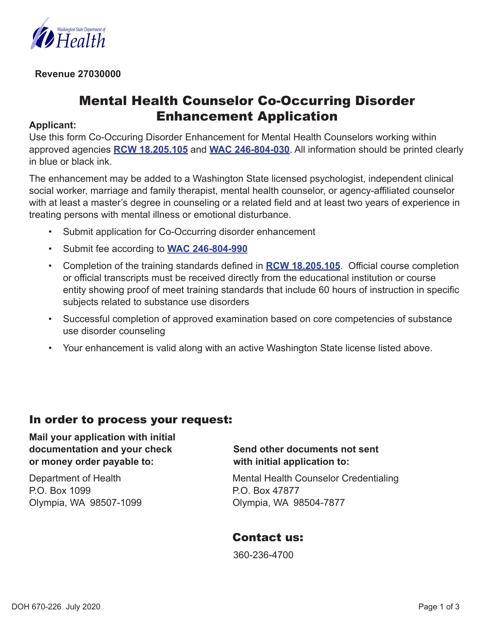**Detailed Caption:**

The image is a detailed screenshot of an official document, predominantly featuring black text on a white background. In the top left corner, there is a logo with unreadable text beside the prominently displayed word "Health" in blue. Below the logo, in black text, the revenue figure "$27,030,000" is noted. 

Centered at the top of the page, the bold black heading reads "Mental Health Counselor Co-Occurring Disorder." Below this, the subheading "Enhancement Application" can be found, followed by a clarifying sentence stating, "Applicants use this form for the co-occurring disorder enhancement for mental health counselors working within approved agencies." In blue text, the document references specific codes: "RCW 18.205.105" and "WAC 246.804.030."

The next paragraph, in black text, instructs that all information should be printed cleanly in blue or black ink. It explains that the enhancement can be added to Washington State licensed professionals such as psychologists, independent clinical social workers, marriage and family therapists, mental health counselors, or agency-affiliated counselors who hold at least a master's degree in counseling or a related field and possess a minimum of two years' experience treating individuals with mental illness or emotional disturbance.

Two bulleted items follow, though they are not detailed in this summary. At the bottom, a bold notice states, "In order to process your request," followed by further directions concerning the submission of additional documents not sent with the initial application. 

The document provides a contact number in bold: "360-236-4700." At the lower left corner of the page, the code "DOH 670-226-July-2020" indicates the document version and date. The bottom right corner specifies the pagination, noting "Page 1 of 3."